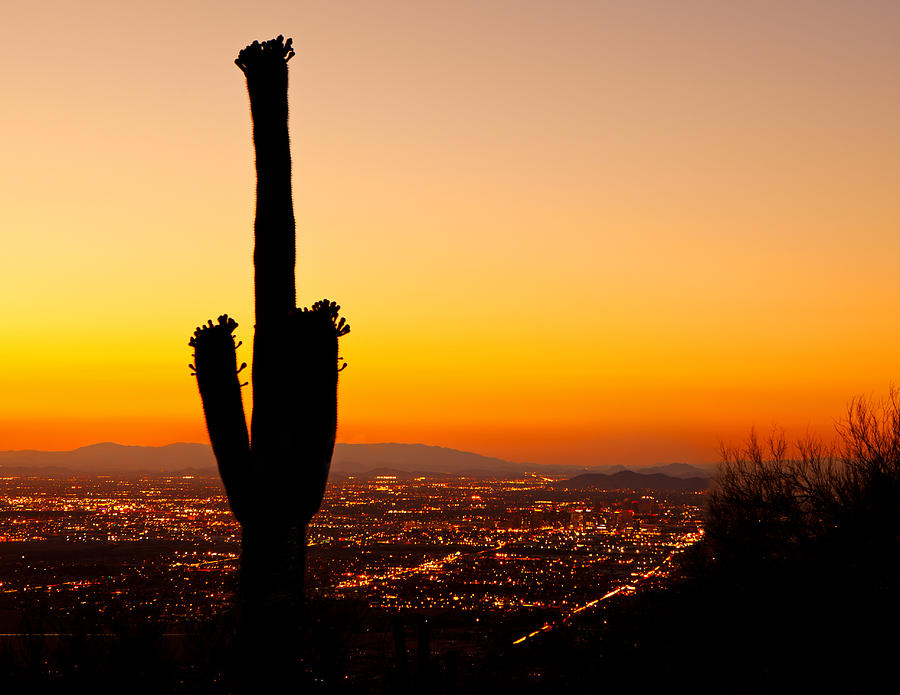A breathtaking sunset paints the sky with a gradient of colors, starting with deep orange at the horizon, transitioning into yellow, and finally fading into a light gray. In the foreground, a dark silhouette of a cactus stands prominently, barely visible against the backlight of the setting sun. To the right, sparse bushes add texture to the desert landscape. Below the sky, a sprawling city comes to life with twinkling lights lining the highways, possibly suggesting a major metropolitan area like Denver or Phoenix. In the backdrop, a majestic mountain range stretches across the horizon, with peaks gradually tapering off to the right. The scene beautifully captures the tranquil yet vibrant transition from day to dusk in the American West.